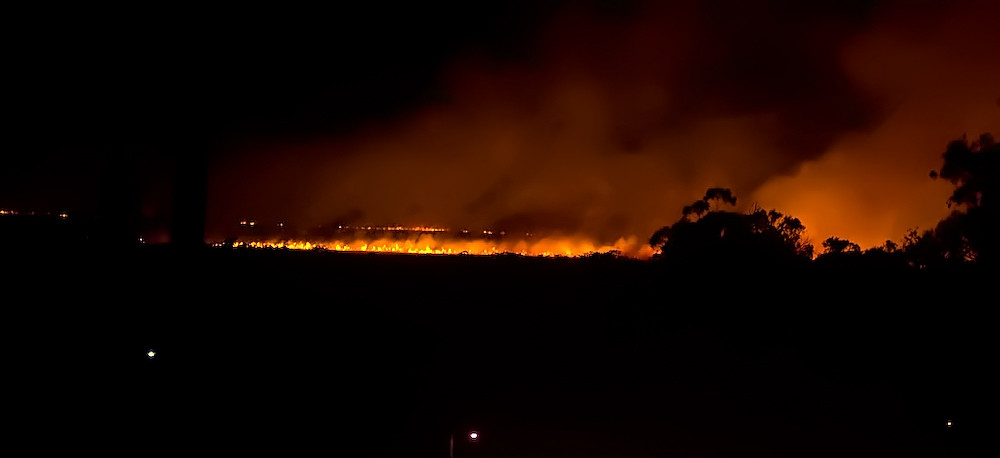This panoramic nighttime image captures a distant forest or brush fire, illuminating an otherwise dark landscape. The bright, glowy orange flames are low to the ground, suggesting a widespread grass fire that has yet to reach a line of trees or bushes discernible in the foreground. Smoke billows upward from the blaze, shrouding the sky with a thick haze. The contrast of the fire’s intense orange and yellow hues against the deep black of the night sets a dramatic scene. Specks of light can be seen across the dark field, adding depth to the composition. There is no text in the image. The overall setting appears isolated and under the cover of night, with the fire providing the only light source, hinting that this moment could be captured in the early morning or late at night.